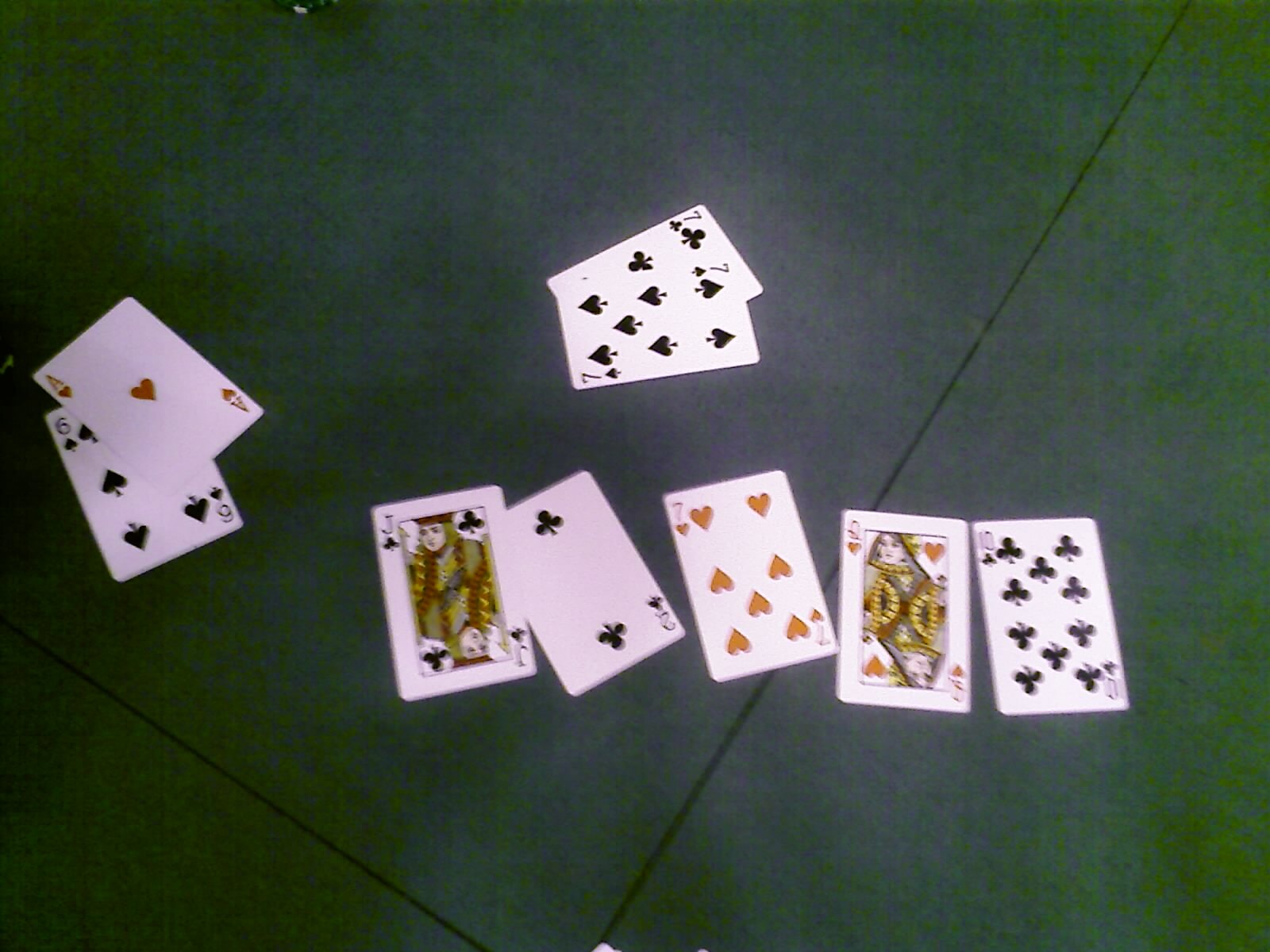The photograph depicts several playing cards scattered on a flat, grey slate-colored surface that appears to be flooring or tiling rather than a table. The surface, featuring discernible lines that suggest individual tiles or pieces of flooring, serves as the backdrop for the cards. The cards are not part of a complete deck but are arranged haphazardly, potentially indicating they were discarded during a game or simply dropped. The cards are grouped in pairs, with a six of spades and an ace of hearts overlapping, a seven of clubs and a seven of spades stacked together, a jack of clubs near a two of clubs, and a seven of hearts beside a queen of hearts. Additionally, a ten of clubs is positioned next to the queen of hearts. The image contains no text.